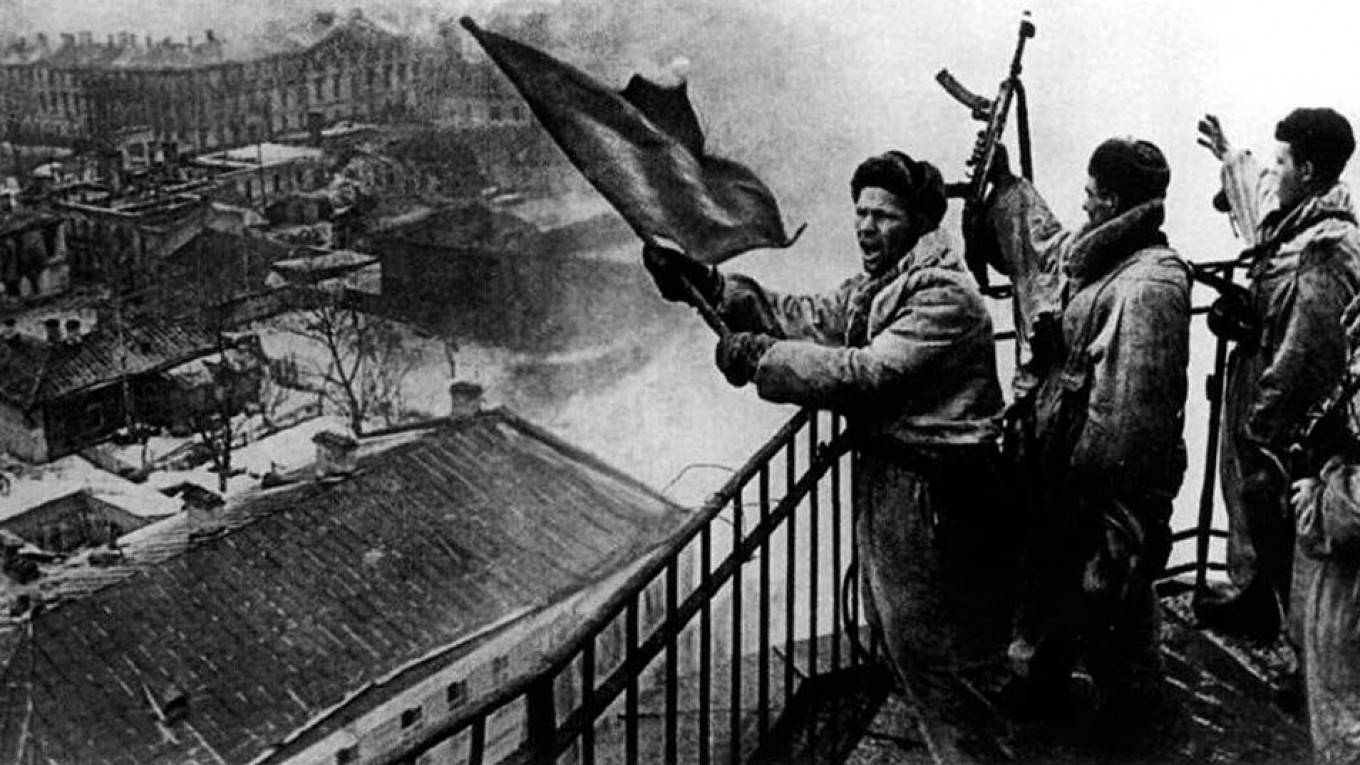This black-and-white photograph captures a moment of apparent celebration, possibly following a military victory, taking place on a foggy day. Three soldiers in heavy jackets and pants stand on a metal-railed balcony, located at the bottom right of the composition. The man furthest to the right has his right arm raised into the air. The middle soldier prominently holds an automatic rifle, resembling an AK-47, aloft. The soldier on the left waves a flag back and forth, suggesting a gesture of surrender or victory. The balcony overlooks a seemingly desolate cityscape with various buildings and houses stretching across the left and upper parts of the image. The city appears almost abandoned, with trees either barren or only partially leafed. Notably, in the background, a large, castle-like structure with numerous windows punctuates the scene, shrouded in mist, adding to the historical ambiance of the photograph.